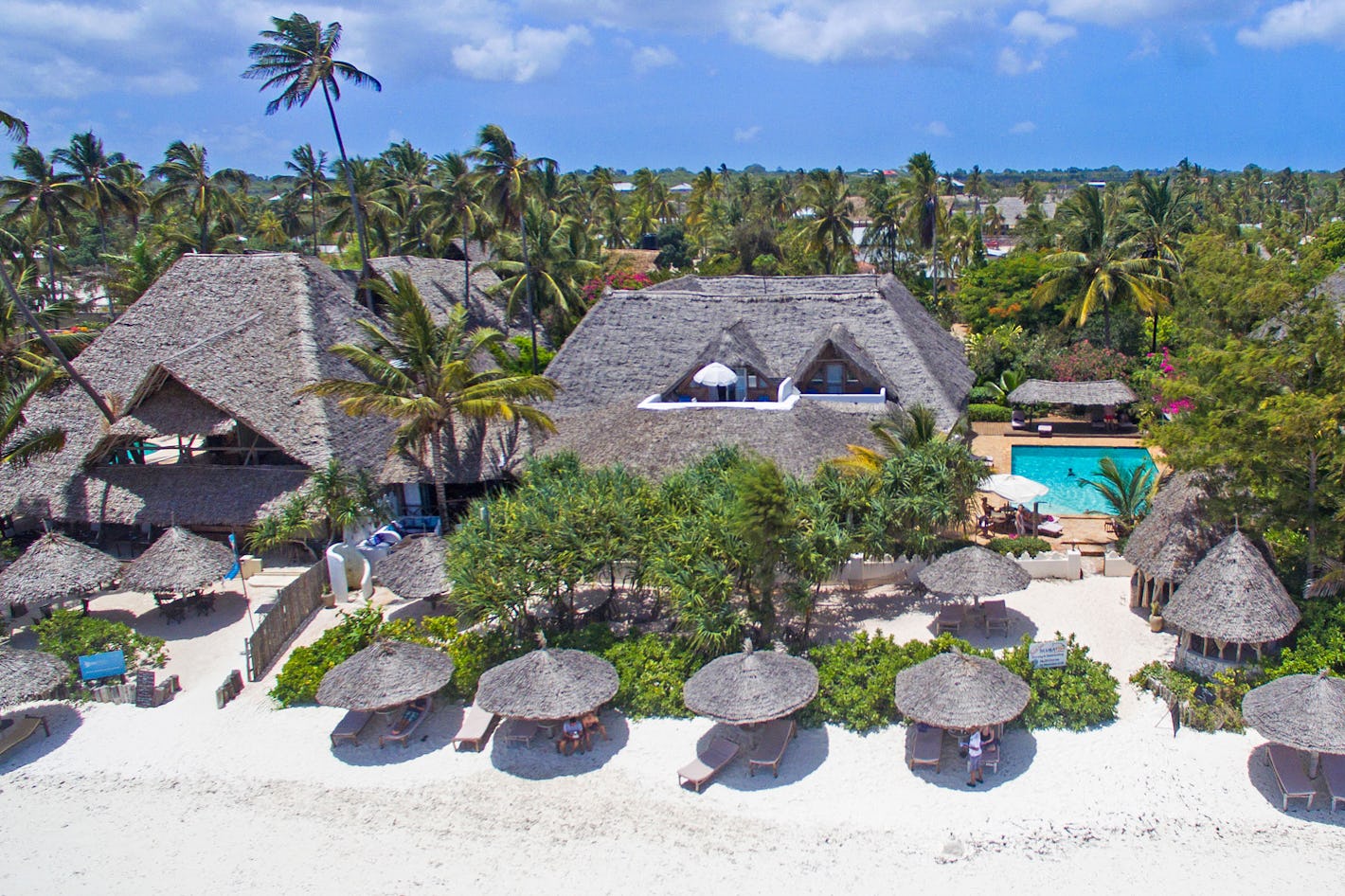This is an aerial view of a serene beachfront vacation resort, bathed in the clear, bright light of a sunny day with minimal clouds. The ground is covered in pristine white sand reminiscent of tropical paradises such as Mexico or the Caribbean. Numerous green palm trees dot the landscape, adding to the lush, relaxing atmosphere.

Prominently featured are five beach umbrellas with dark gray, cone-shaped thatched roofs providing shade to several tiny, indistinct figures lounging beneath them. A striking rectangular pool filled with bright blue water stands out in the middle of the scene, adding an inviting splash of color.

In the background, several beach houses or cottages can be seen, particularly a notable house on the right side with a square flat roof, featuring two upright triangular exterior pieces that suggest the presence of porches. The overall sense is one of tranquility and relaxation, an ideal spot for a peaceful getaway.